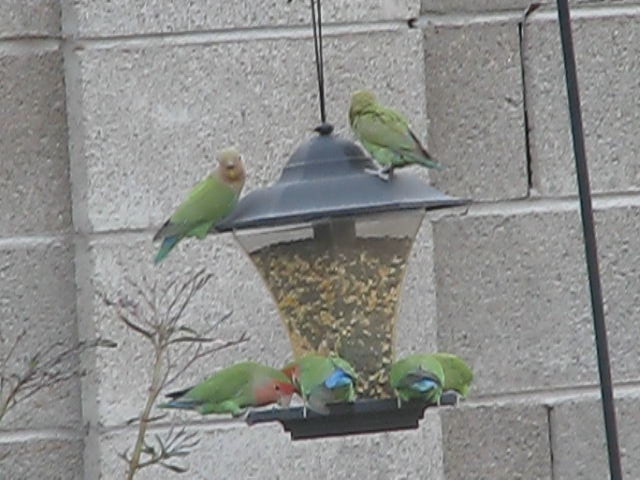The photograph, taken outdoors, features a bird feeder hanging from a black string in front of a gray, cinderblock wall. The feeder has a clear house filled with light brown, tan, and dark brown seeds. Its UFO-shaped top, where two green parakeet-like birds are perched, contrasts with the black ledge at the bottom where three other parakeets are feeding. One of the feeding birds has a red face, while the others have blue and black tails, adding vibrant splashes of color. Bare branches frame the left side of the image, and an iron rod or stake is visible on the right, supporting the feeder. Additionally, a plant can be seen in the left-hand corner, contributing to the natural setting.